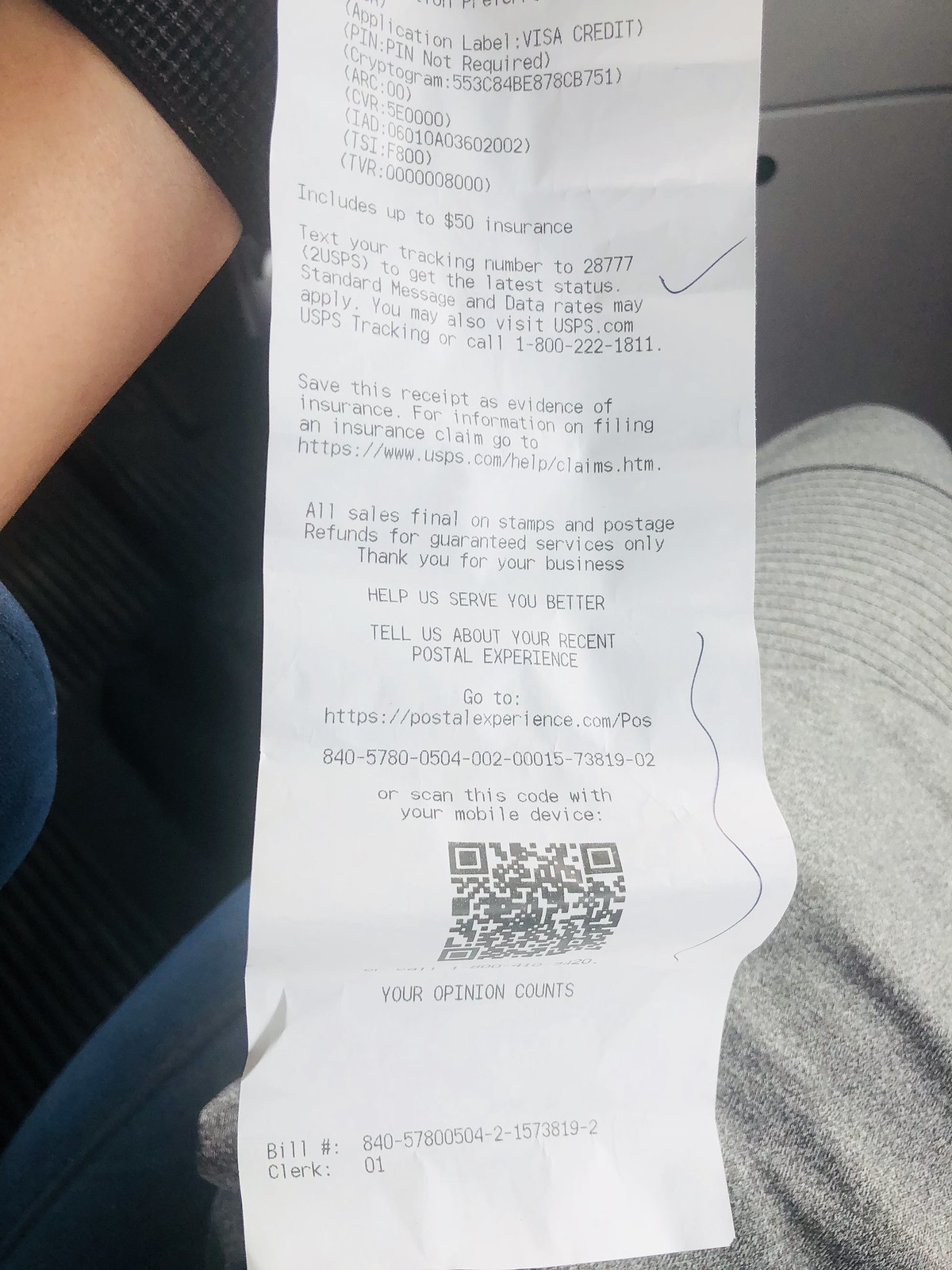A detailed and comprehensive photograph depicts an individual sitting inside a car, holding up a long receipt from their most recent purchase, likely from a post office. The person’s gray pants and knee are visible beneath the receipt, with part of their wrist near the top left of the image. The receipt, held against the car's interior, shows detailed transaction information, including "application label," "visa credit," and "PIN not required." There's a cryptogram accompanied by a series of letters and numbers, and a section confirming the inclusion of up to $50 of insurance. 

Additional details on the receipt offer guidance on tracking packages via text to 28777 or through USPS's official website or customer service number. Noticeably, it emphasizes the importance of saving the receipt as evidence of insurance and offers information on how to file an insurance claim on the USPS website. The bottom of the receipt contains a URL for a customer feedback survey and a QR code for easy access. A check mark and a long scribble are also visible, along with a bill number and a clerk number. The setting inside the car is evident from the visible car mat and part of the dashboard, giving a sense of the environment in which the photo was taken.